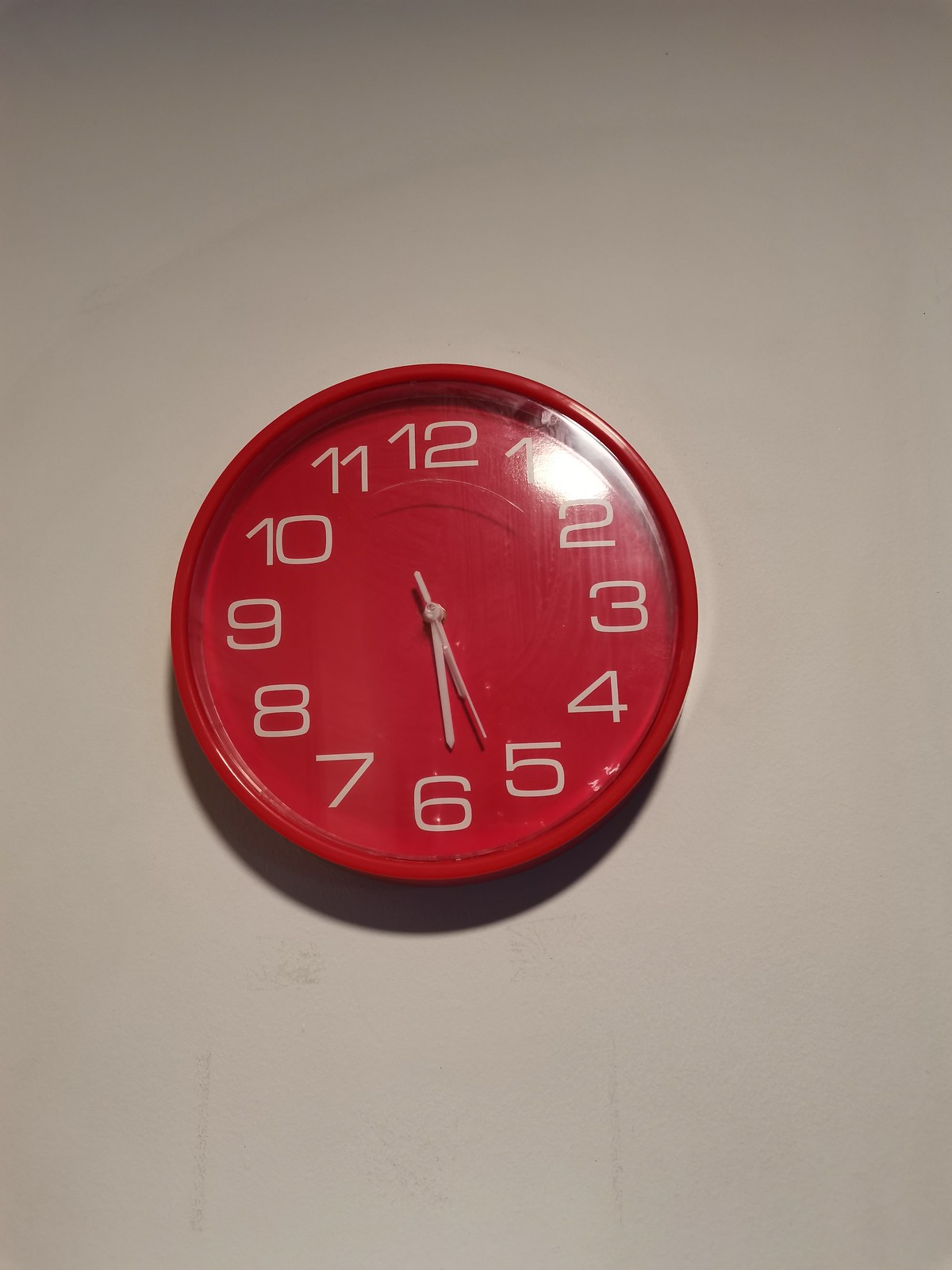The image depicts a bright red, circular wall clock with white Arabic numerals, mounted on a white wall. The clock features white hour, minute, and second hands, with the time showing approximately 5:26 or 5:27. The clock face, which appears to be made of paper or cardboard, has no hash marks between the numbers. The frame of the clock is red plastic, potentially with a clear perimeter allowing partial visibility through it. There is a noticeable glare from a ceiling light fixture reflecting off the plastic surface, suggesting the clock's glass is likely plastic rather than glass. The clock casts a slight shadow on the wall, indicating the light source is nearby. Overall, the clock has a somewhat cheap appearance but adds a colorful touch to the otherwise plain white wall.